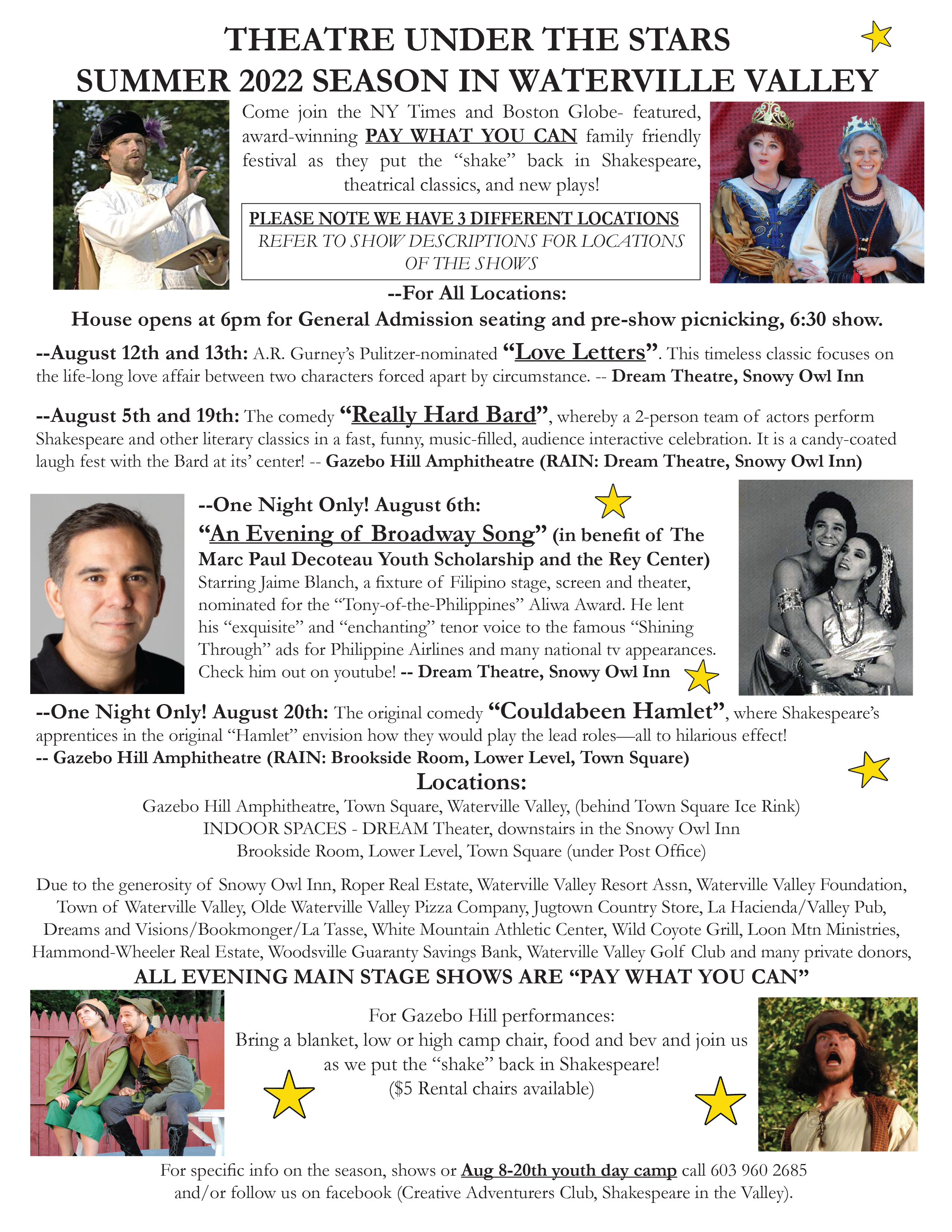The image is an advertisement flyer for the "Theater Under the Stars" Summer 2022 season in Waterville Valley. The flyer prominently features the text "Theater Under the Stars, Summer 2022 in Waterville Valley" in black font at the top. Below this, the flyer has a mix of descriptive text and visuals. 

On the left side, there is a photo of a man wearing a black school cap and a white long-sleeved shirt, appearing to act while holding a book in his right hand. Directly to the right side, two women are adorned in fairy-tale princess outfits; the younger woman has brown fluffy hair and wears a gold crown, while the older woman has gray hair with a silver crown. Further down, on the left, there is an image of two men dressed like Robin Hood sitting on a bench, while on the right, a man in medieval attire appears to be screaming. There is also an image of a middle-aged man and another of a couple dressed in Sinbad or Aladdin-style outfits hugging. 

The flyer highlights the season's schedule with events such as "Love Letters," "Really Hard Barred," a one-night performance of a comedy (potentially Hamlet), and "An Evening of Broadway Song" set for August 6th. The text also notes that all evening main stage shows follow a "pay what you can" policy. The events are held at the amphitheater, located in the town square of Waterville Valley.